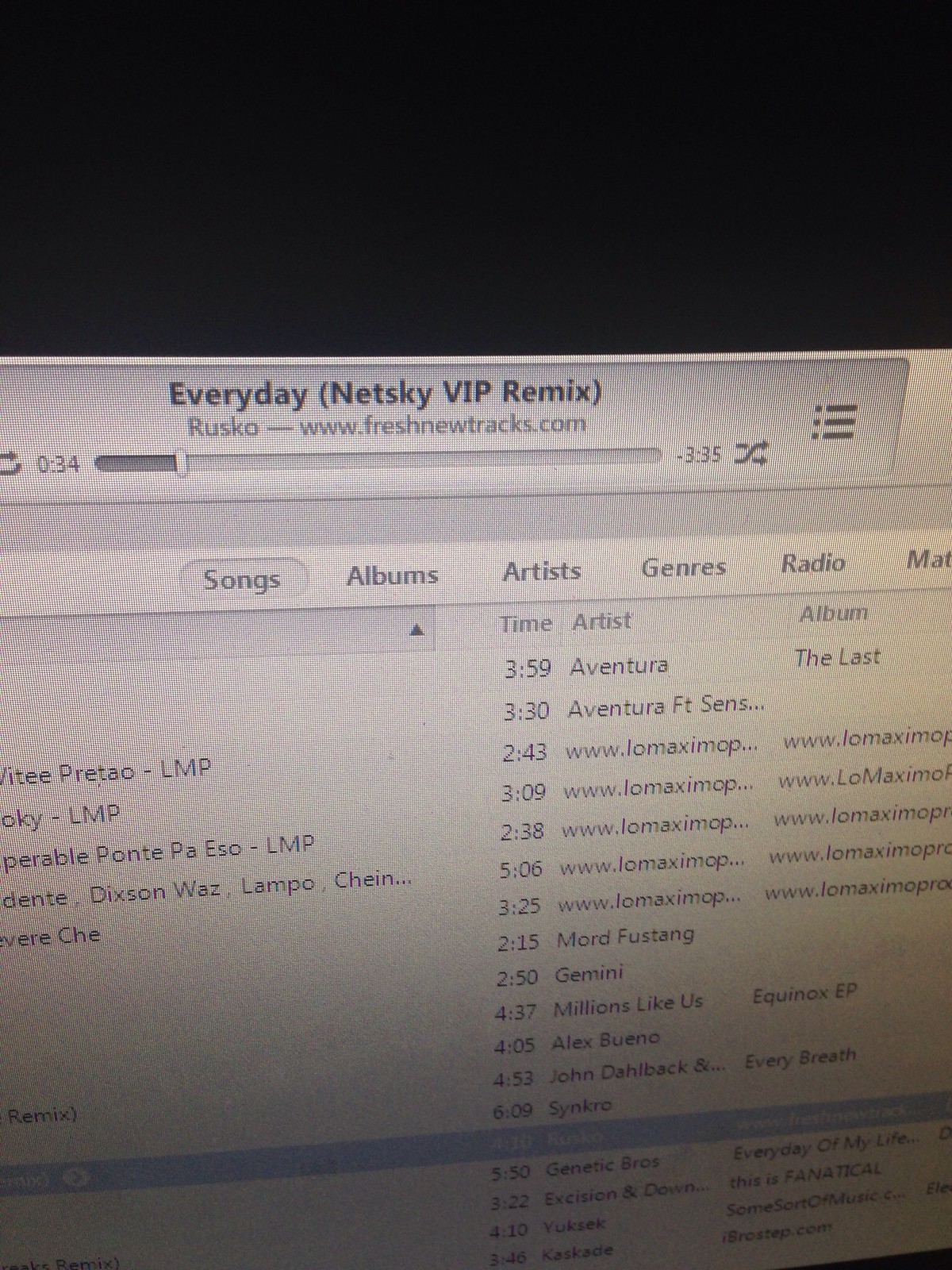The image is a grainy and low-light photograph of a rectangular computer screen, likely displaying an older version of iTunes. The screen appears dim, suggesting the picture was taken in the dark. At the top of the screen, we can see the iTunes Player with control buttons and a progress bar, indicating a song is playing. The song title "Every Day (Netsky VIP Remix)" by Rusko is displayed along with a timestamp showing 34 seconds played out of a total of 3 minutes and 35 seconds.

Beneath the player controls, there are various headings such as "Songs," "Albums," "Artists," "Genres," and "Radio," suggesting the organizational layout of the playlist. The background of the screen is white, lending a modern, almost futuristic feel. Despite the poor image quality, several song and artist names can be discerned, including "Gemini," "Millions Like Us," "Equinox EP," "Alex Bueno," "John Dahlback," and "Synchro."

Nearer the bottom of the display, a song is highlighted, indicated by a blue selection bar, though its details are faded and hard to read due to the graininess and lighting conditions. Additionally, the screen exhibits a cross pattern, typical of a photograph taken directly from a digital display, contributing to the overall poor clarity of the image.